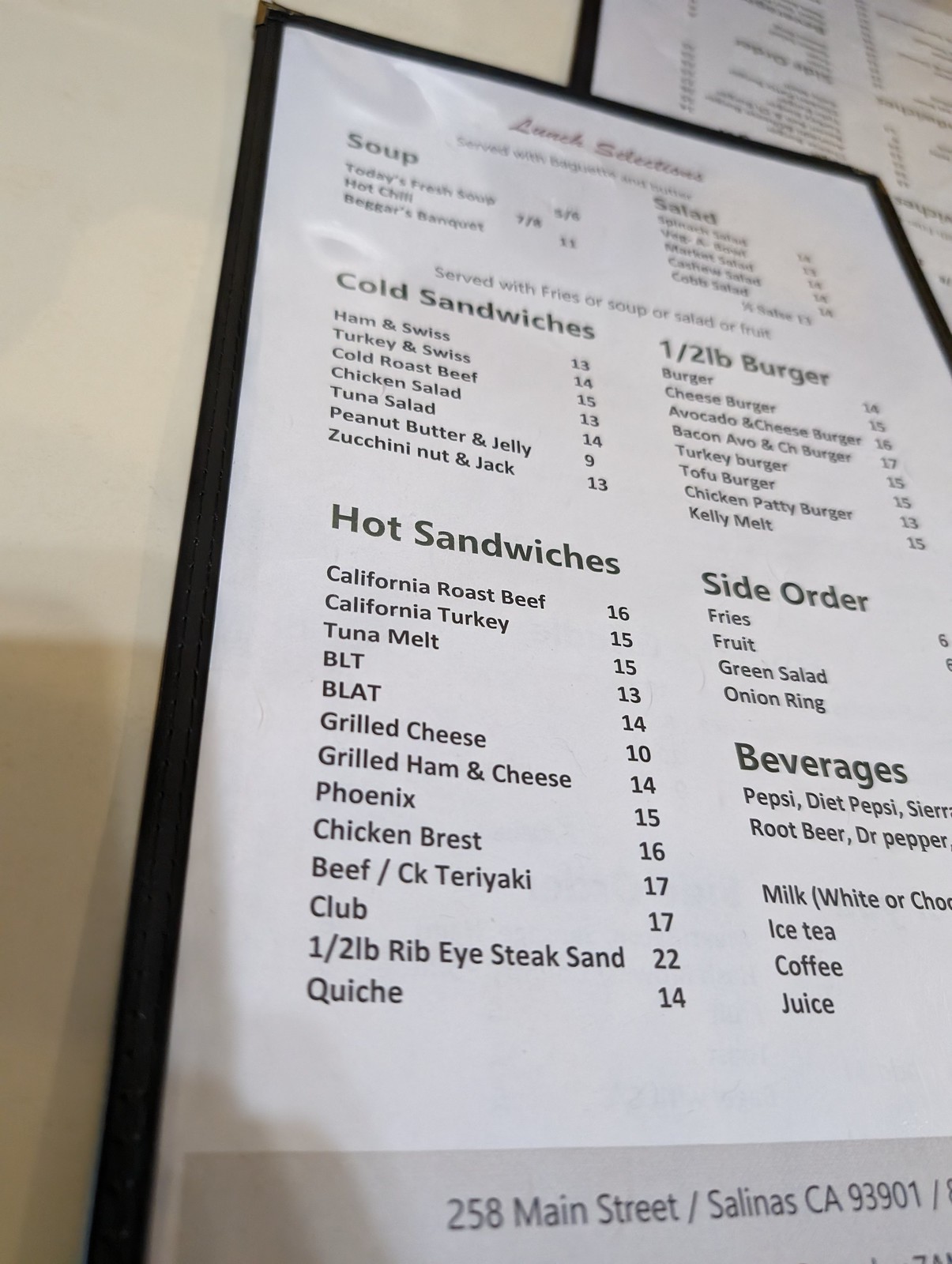The image is a photograph of a restaurant menu taken from an angled perspective. The overall shape of the photograph is rectangular, with the top and bottom sides being half the length of the left and right sides. The menu itself is also rectangular, encased in a clear plastic holder with black fabric edges and silver corner caps on all four corners. Due to the angle of the photograph, part of the menu is out of frame on the right, and it appears larger towards the bottom than at the top. Additionally, the menu is slightly tilted towards the left.

The menu rests on a cream-colored table surface, and another identical menu is placed underneath it, upside down and opposite in orientation. The menu features multiple lines of black text on a white background. The legible text at the top reads, "Lunch Selections," followed by categories such as "Soup," "Today's Fresh Soup," "Hot Chili," and "Beggar's Banquet." The text then transitions to "Salad," but the remainder of this section is mostly blurry and out of focus, rendering it illegible.

Further along, the menu lists items under the header "Served with Fries or Soup or Salad or Fruit," followed by "Cold Sandwiches." The sandwich options include "Ham and Swiss, 13," "Turkey and Swiss, 14," and "Cold Roast Beef, 15."